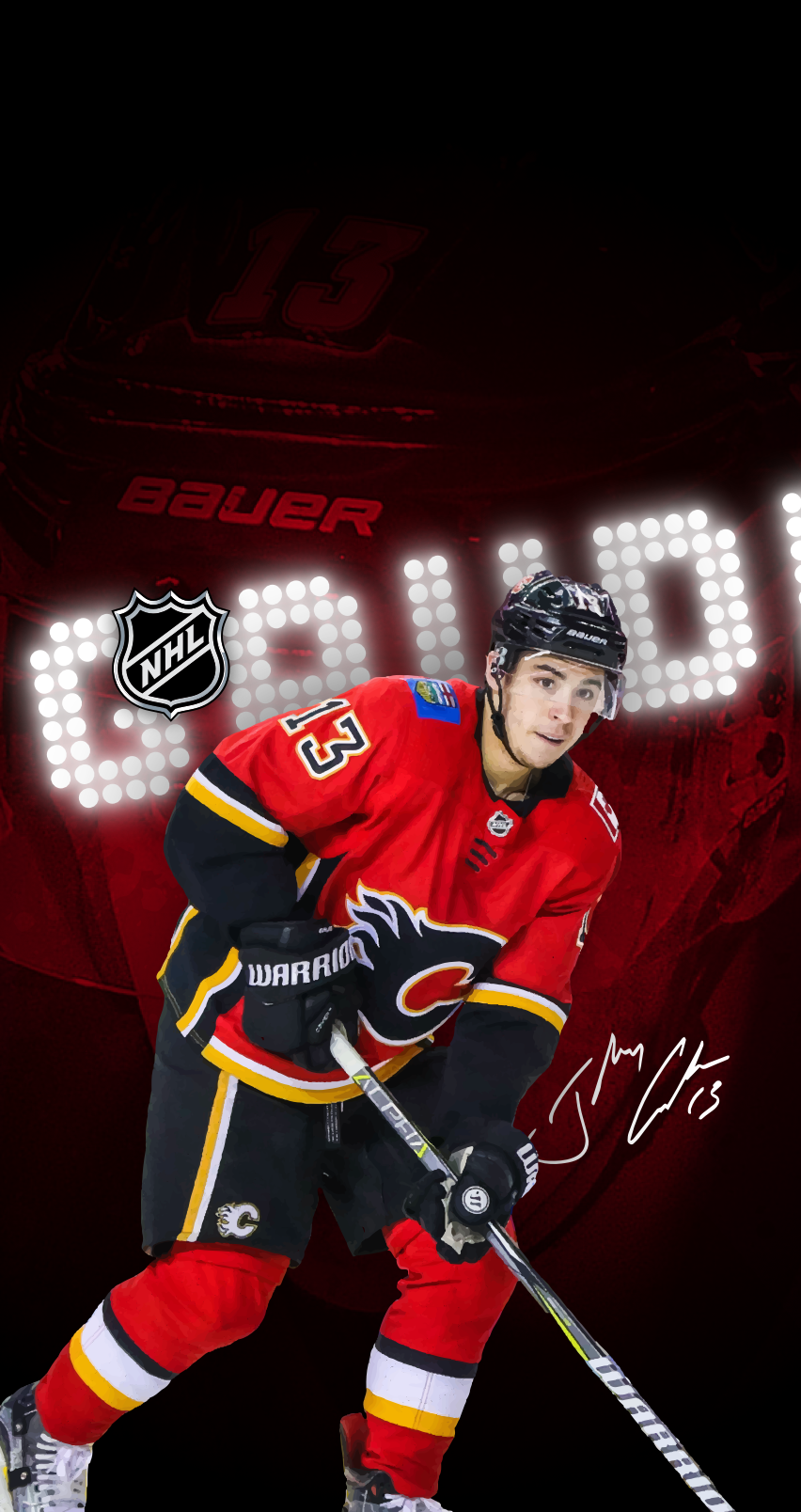This image depicts a young NHL hockey player in full gear, wearing the number 13 jersey with his last name, Bauer, prominently displayed. The player, appearing to be no older than 30, is shown in an action shot, likely intended for a player card or professional profile. He is clad in a red top jersey with black accents and sleeves, black gloves—one embossed with "Warrior" in white—and black pants featuring yellow and white stripes. His outfit also includes black and white ice skates and a black helmet with a clear protective visor. Notably, he holds a hockey stick as if actively engaged in play, focused on something outside the camera's capture. The background of the image is red with the number 13 and the name Bauer written in white at the top. Additionally, the NHL emblem is present on the left side of the image, signifying its professional nature. The player's dark brown eyes and mouth guard contribute to his intense and concentrated look.